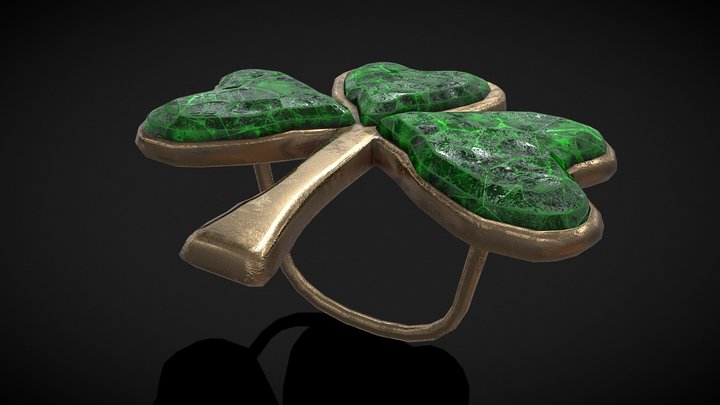The image is a colored, artistically staged photograph, taken indoors against a simple, black background. The focus is on a ring designed in the shape of a three-leaf clover. The ring's band and setting appear to be made of a dull, brass-like metal, possibly gold, although it lacks the characteristic shine. The clover itself is composed of three heart-shaped green stones, each displaying an intricate pattern of green and black hues with varied brightness and darker veins running through them. This detailed texture gives the stones a unique, non-shiny appearance. The ring is positioned with the band facing downwards, balanced delicately on its edge, casting a subtle shadow towards the center left of the image. The entire scene is photographed from an up-close perspective, emphasizing the fine details of the ring and its stones.